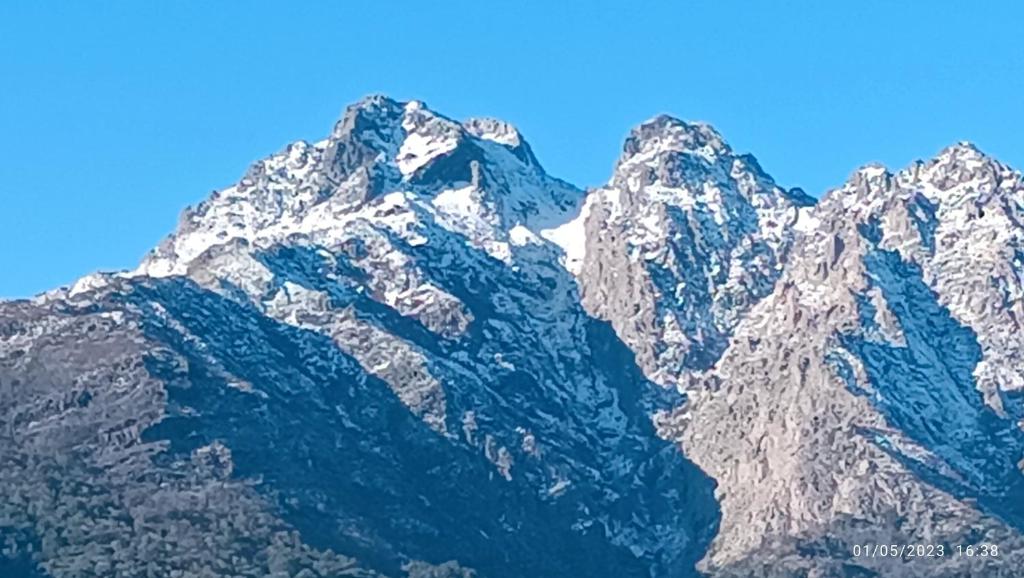The image captures a stunning outdoor scene featuring a steep, imposing mountain range, possibly located in Chile. The peaks of the mountains are predominantly composed of gray rock with patches of snow, highlighting their rugged beauty. The clear blue sky above contrasts sharply with the rocky terrain below, indicating it was taken on a bright, sunny day. The well-lit surroundings add a vibrant clarity to the image. A shadowed valley to the left is noticeable, providing depth and dimension, while sparse vegetation clings to the lower sections. The photograph, rich in detail and color, also contains a timestamp in the bottom right corner, reading "January 5th, 2023 at 1638 hours," yet no other text is present. The high-definition quality of the image suggests it was captured by a skilled nature photographer, emphasizing the majesty and serene beauty of the mountainous landscape.